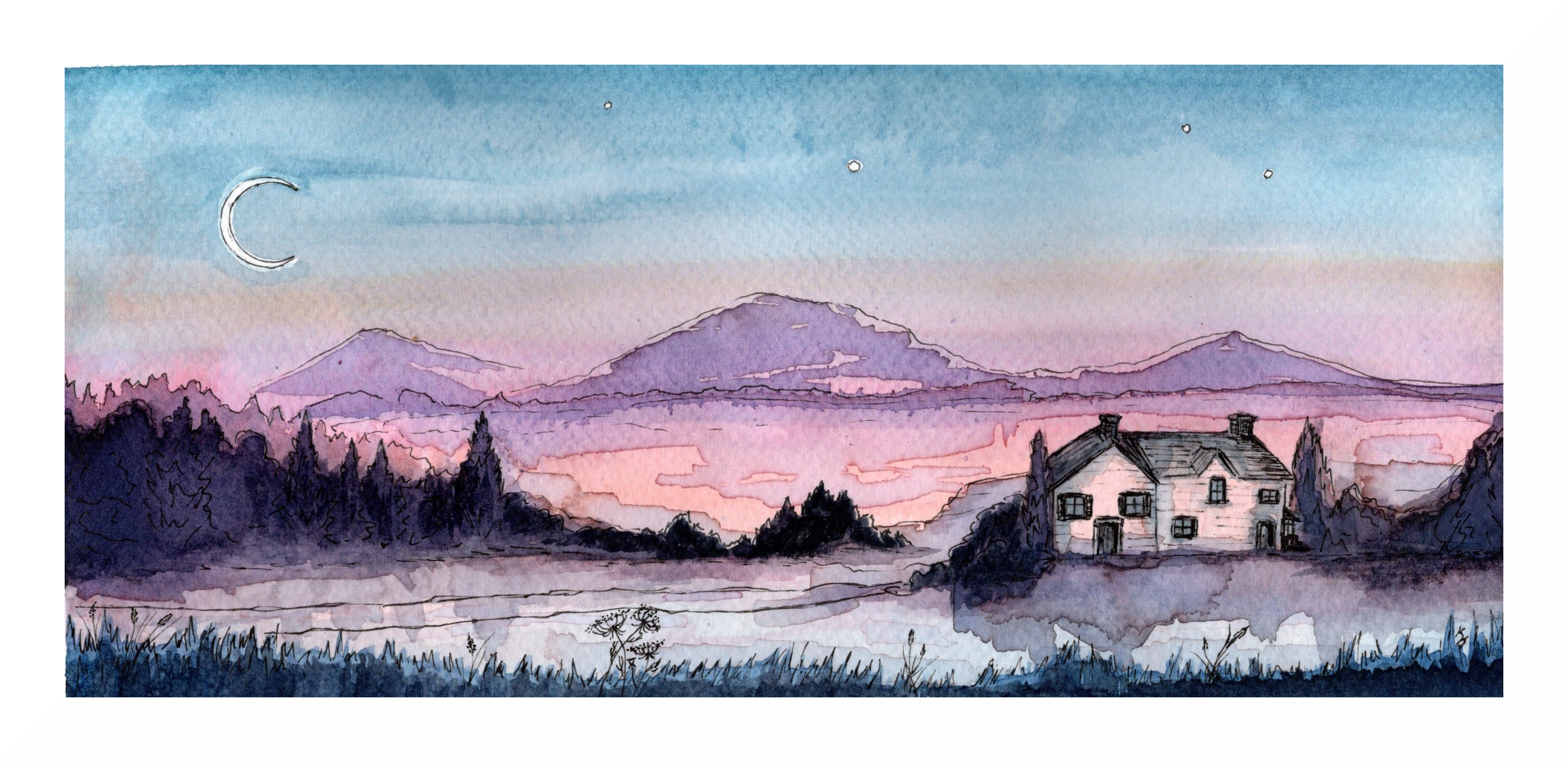This is a detailed watercolor landscape painting characterized by a horizontal, panoramic format, wider than it is tall. The scene portrays a tranquil nighttime view dominated by a harmonious blend of blue, purple, pink, and some golden tones, creating a gradient that accentuates the fluid, granulated texture of the paint. 

The sky features a light blue wash at the top, transitioning into softer golden hues near the horizon. A thin crescent moon, along with several scattered stars, illuminates the left-hand side of the sky. Below the sky, a range of purple mountains spans the background, their peaks gently outlined against the colorful heavens.

Nestled in the valley at the base of these mountains, which may also reflect in a possible lake or waterway rendered in pinkish hues, sits a lone, wide, white farmhouse. This house, positioned on the right side, is accented by a dark roof, multiple windows, and two chimneys. Flanking the house are tall, vertical cedar trees, adding a touch of greenery to the scene.

The foreground is detailed with dark green and coniferous trees towards the left, transitioning into a mix of shrubs and vibrant grass along the bottom edge. Flowers speckle this grassy area, adding subtle, colorful highlights to the painterly landscape.